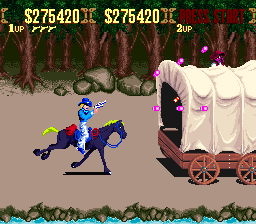This is a detailed screenshot from a vintage pixel art video game, possibly from a classic console like the Nintendo NES. The scene depicted is a western chase where the protagonist, a cowboy in blue attire including a blue shirt, pants, and hat, rides a dark blue horse with a red saddle. The cowboy wields a pistol in his right hand, pursuing a brown wooden covered wagon with a white top, visible on the right side of the image. Atop the wagon, there's another cowboy with a mask and pink bullets flying towards the right, indicating active gameplay.

The background features a landscape with trees and rocks at the top, and a trail with a water edge at the bottom. The game's user interface, displayed at the top of the screen, shows scores and lives: "1 UP" indicating the active player, who currently has $275,420 and three lives left represented by three gun icons. "2 UP" prompts for a second player to join with "Press Start," implying the game supports multiplayer mode but currently only one player is engaged.